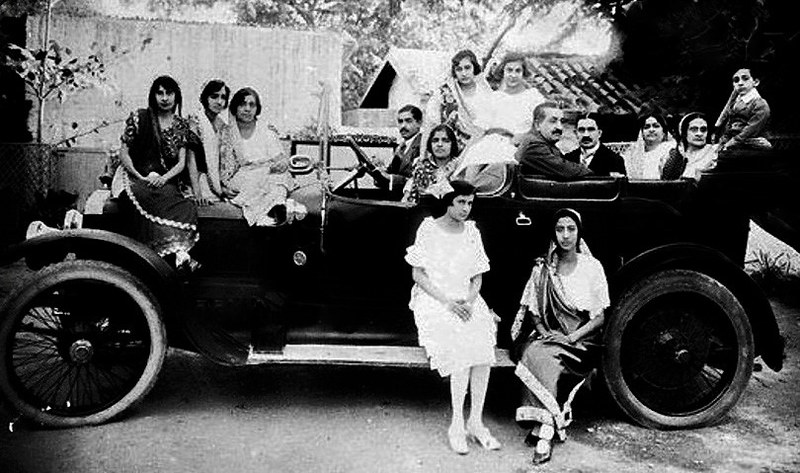This early 20th-century black-and-white photograph captures an Indian family during what appears to be a joyous celebration, possibly a wedding or family gathering. The centerpiece of the image is a large, open-top Model T-style car, which showcases its distinct, skinny tires with thin spokes and silver-striped detailing around the door and windshield. The car is filled to capacity, with over a dozen people occupying every available space: some seated in the front and back seats, others perched on the hood, fender, and running boards. The men, many with dark hair and some sporting mustaches, are elegantly dressed in suits. The women, also dark-haired, are adorned in dresses or robes. The background features a stone wall and glimpses of a building with a peaked roof and surrounding trees, suggesting an outdoor setting. The overall atmosphere is one of enjoyment, with the family members cheerfully basking in the sunlight, their faces embodying the spirit of celebration.